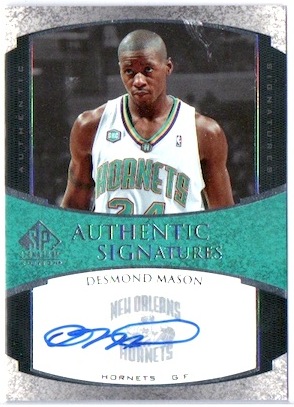The image is a professionally designed, portrait-oriented basketball trading card featuring Desmond Mason of the New Orleans Hornets. The card has a silverish border at the top and bottom, framing the central image of Mason, an African American basketball player wearing a white Hornets jersey with the number 24. The player is positioned directly in the center of the card and is looking up to the left.

Across the bottom part of the image, there's an aqua-colored band with a diamond-shaped logo on the left that reads "SP" followed by the text "Authentic Signatures." Beneath this banner, within an arc-shaped white rectangle, is the name "Desmond Mason" and the New Orleans Hornets logo in light green. The card also features Mason's blue ink signature. The colors used include white, black, gray, blue, light blue, green, brown, different shades of gray, and silver. The overall design and presentation emphasize its status as a collectible, showcasing both photographic and textual elements in an elegant and structured format.